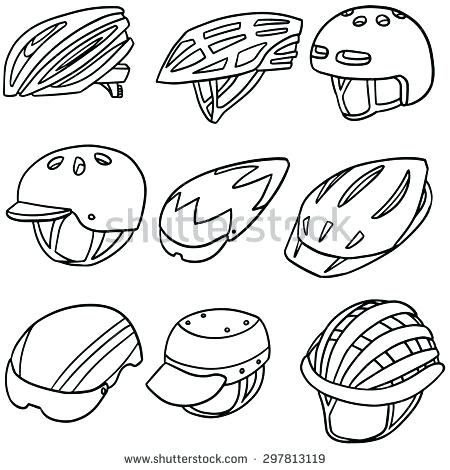The image shows nine distinct bicycle helmets arranged in a 3x3 grid pattern on an all-white background. Each helmet is depicted in black and white as detailed line drawings. The variety of helmets includes different shapes, such as round, triangular, slim, and dome-like designs. Some helmets feature front visors, slits, or holes for ventilation, while others have solid tops or striations across the surface, as well as chin straps. The middle of the image features a gray Shutterstock watermark, and at the bottom, the text www.shutterstock.com-297813119 is also in gray.